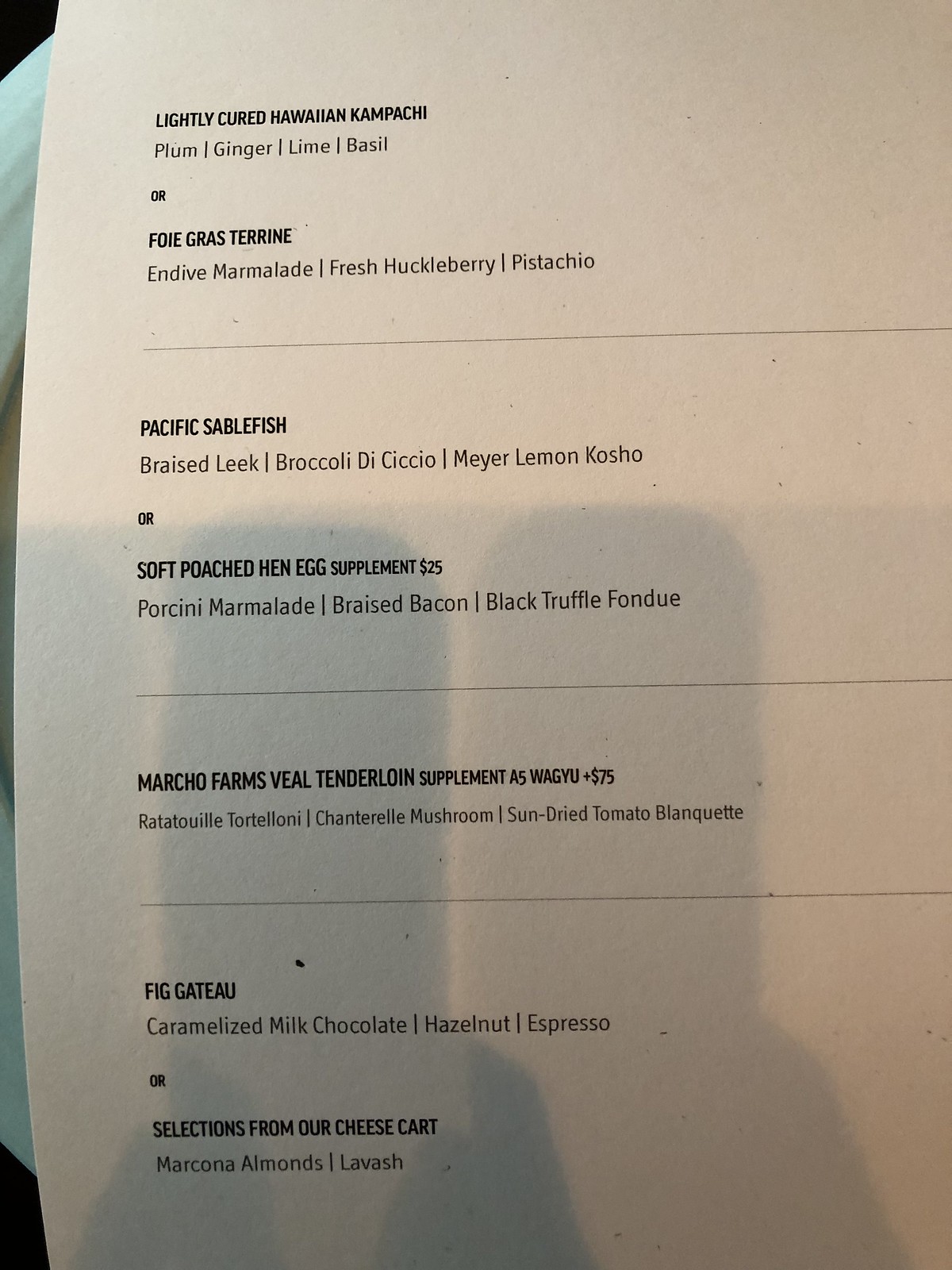**Description:**

An indoor color close-up photograph of a simple menu printed on plain white paper. The menu items are listed in dark black ink and includes the following detailed descriptions:

- **Lightly Cured Hawaiian Kampachi**
  - Plum, Ginger, Lime Basil
- **Foie Gras Terrine**
  - Endive Marmalade, Fresh Huckleberry, Pistachio

A thin horizontal line separates the sections.

- **Pacific Sablefish**
  - Braised Leek, Broccoli de Cicco, Meyer Lemon Curd
- **Soft Poached Hen Egg (Supplement: $25)**
  - Bacon Marmalade, Braised Bacon, Black Truffle Fondue

Another thin horizontal line divides these items from the next section.

- **Marcho Farms Veal Tenderloin (Supplement: $75)**
  - A5 Wagyu, Tortellini, Chanterelle Mushroom, Sun-Dried Tomato Blanket

The final line item:

- **Fig Tart**
  - Caramelized Milk Chocolate, Hazelnut, Espresso or Selected from Our Cheese Cart
  - Macaron, Almond Lavash

There is a notable shadow in the lower part of the image, reflecting the hands of the person who took the photograph with their cell phone. The shadow of the hands is clearly visible, adding a personal touch to the otherwise stark and simple menu presentation.